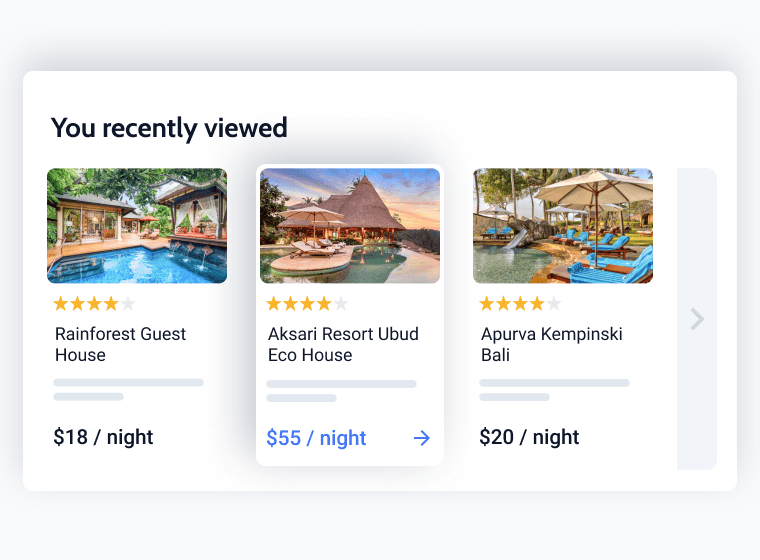This is a cropped screenshot of a travel website, likely Expedia, showcasing a section titled "You Recently Viewed" located at the top left, displayed in black text on a white background. The section features three vertically oriented rectangular boxes aligned side by side, each highlighting different accommodation options.

The first box presents the "Rainforest Guesthouse." At the top of the box, there is a thumbnail image depicting the pool area. Below the thumbnail, a star rating indicates a score of 4 out of 5 stars. At the bottom, the nightly rate is shown in black text, stating "$18 a night."

The second box follows a similar layout, with a thumbnail image at the top and a star rating positioned just below the thumbnail to the left. The name of this accommodation is displayed, and the nightly rate, "$55 a night," is highlighted in blue text with an arrow directing to the right.

The third box also mirrors this format, featuring a thumbnail at the top, a star rating on the bottom left, the name of the accommodation, and a displayed rate of "$20 a night."

To the right of the thumbnails, there is a thin, vertical light blue bar with a gray arrow in the center pointing to the right, suggesting further navigation options.